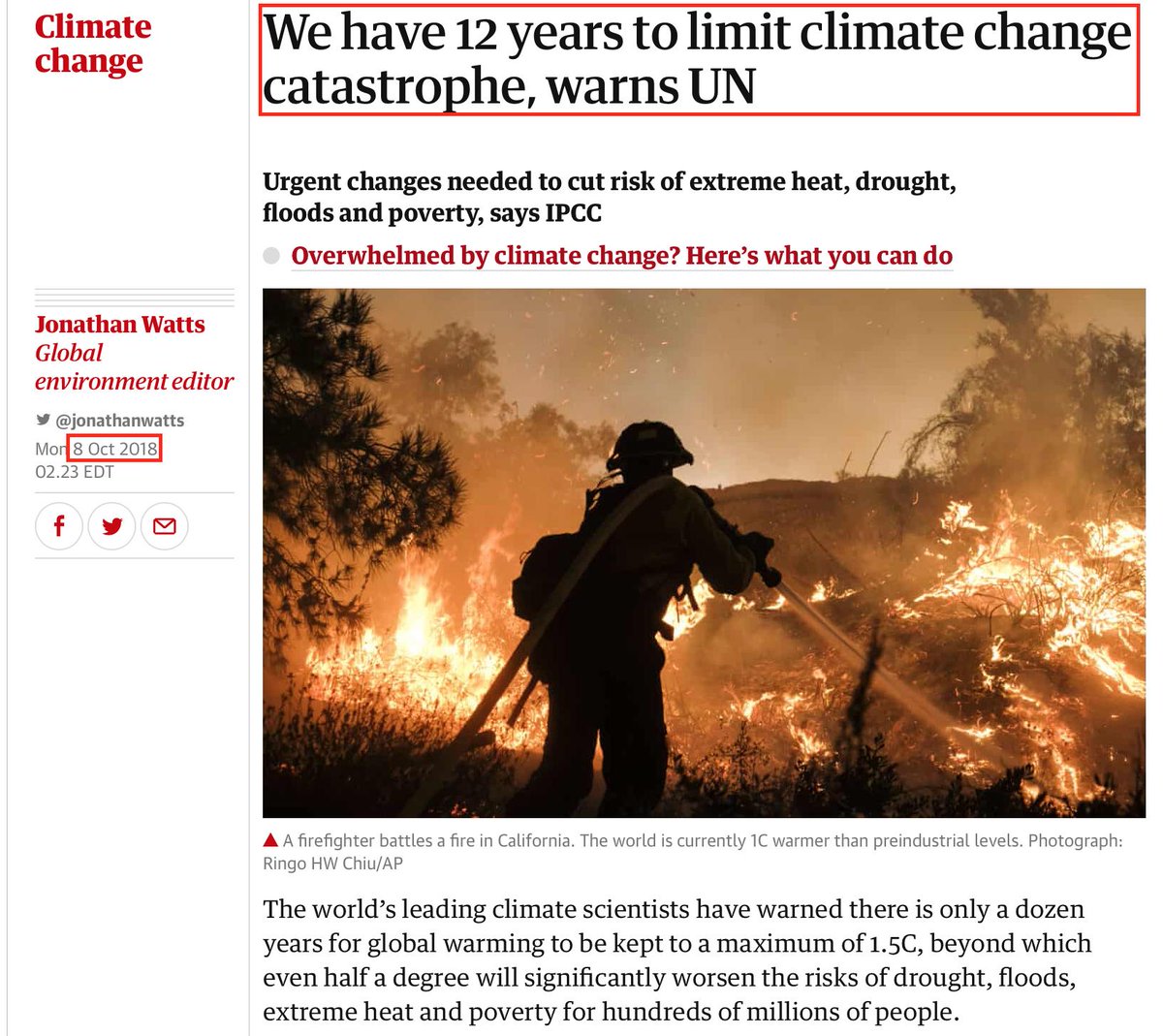In the upper left corner of the image, the text "Climate Change" is prominently displayed in red. Directly below, within a red-outlined square, there is black text that reads: "We have 12 years to limit climate change catastrophe, warns UN." The letters "UN" are capitalized for emphasis. Beneath this, in black text, it says: "Urgent changes needed to cut risk of extreme heat, drought, floods, and poverty, says IPCC," with the letters "IPCC" also capitalized. Just beneath that, the text continues: "Overwhelmed by climate change? Here's what you can do."

The photo, captured at nighttime, depicts a large outdoor area engulfed in flames. Bright yellow fire roars, casting an ominous light. To the left, a lone tree stands, silhouetted against the blaze. In the foreground, the dark silhouette of a firefighter is visible from the back. The firefighter's helmet and protective suit can be distinguished, and he holds a hose that sprays water to the right, battling the relentless inferno.

Below this, accompanied by a triangle icon, the caption reads: "A firefighter battles a fire in California. The world is currently 1°C warmer than pre-industrial levels. Photograph: Ringo HW Chiu-AP." To the left of the photo, encased in a red square, it reads: "Jonathan Watts, Global Environmental Editor." The date, "8th October 2018," is also present in red.